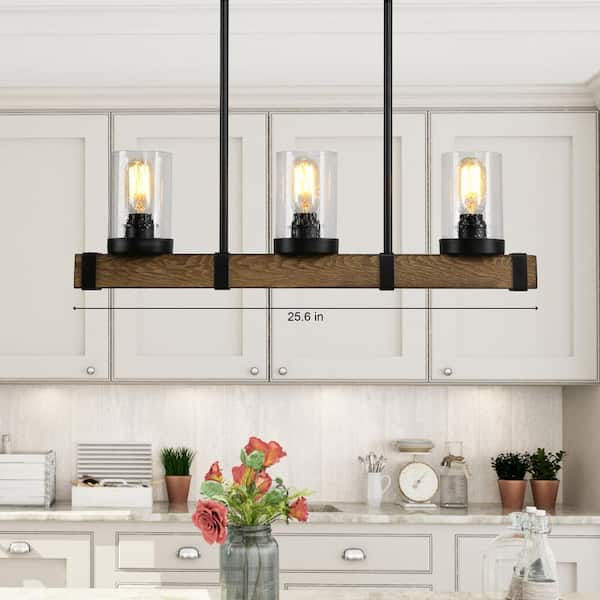The image captures a modern, impeccably clean kitchen characterized by its neutral, ivory, and white color palette. The space is dominated by white marble countertops and white cabinetry adorned with silver handles. Above the counter, a sleek, white backsplash mirrors the cabinetry's pristine appearance. Atop the counter rests a scale, a bottle, and a couple of small clay pots teeming with green plants, likely herbs such as chives. A utensil holder also sits on the counter, contributing to the kitchen’s organizational aesthetics.

Suspended from the ceiling by long black poles, a rustic brown wooden beam features prominently in the room. The beam is highlighted by four black wraps, which secure it to the poles, and supports three vintage-inspired gas lanterns, retrofitted with modern light bulbs encased in clear glass or acrylic housings. These lanterns are designed to mimic a historical aesthetic, complete with black bases and halogen-like bulbs.

A partial view of an island can be seen in the foreground, upon which stands a clear vase with vibrant orange flowers, adding a pop of color to the otherwise neutral-toned environment. This vase of flowers, possibly accompanied by jars of olive oil and vinegar, enhances the kitchen’s fresh, inviting ambiance. The lighting fixture, resembling old-style lanterns, offers a striking contrast to the otherwise contemporary setting, emphasizing the blend of modern and vintage elements that define this kitchen.